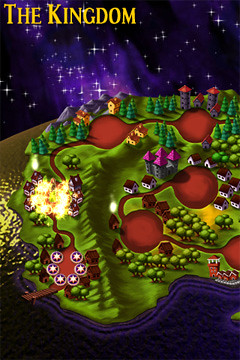"This poster, titled 'The Kingdom,' features an otherworldly landscape that captivates the eye. In the top left corner, the text 'The Kingdom' is prominently displayed in yellow capital letters against a backdrop of vibrant aurora-like lights, which cascade downwards from the upper portion of the image.

The central focus is a globe, possibly representing an alternate world. On the left side of the globe, the moonlight casts a reflective glow upon the water that wraps around this intriguing realm. Brown roads crisscross the landscape, punctuated by several circles which could be parking lots or plazas.

One prominent circle on the left houses six smaller circles, each containing a white star. Leading from this circle is a road that meanders to a small town. This town features three houses on the left – with one notably larger – and three on the right. The central circle of the town is adorned with six yellow lights around its edge and a green and yellow blob in the middle.

Roads extend from this central circle to two other empty circles, one above and one to the right. A further road stretches out and disappears off the edge of the poster.

In the lower section, a half-visible circle connects to more roads and empty circles. Surrounding these are residential structures: two long houses behind, five smaller houses to the right, a castle with a pink roof to the left, and two small houses adjacent to the castle. Nearby, clusters of woods with green, differently-sized circular trees add to the natural beauty. 

Further down, there are five long cabins around another circle and a lighthouse at the bottom right of the poster. In the upper right section of the globe, there are at least two farms featuring alternating silos and houses, complemented by evergreen trees.

To the left of these farms, another circle contains five two-story houses, completing the detailed and whimsical overview of 'The Kingdom.' Below all these land features, the water provides a serene counterpoint to the bustling landscape above."